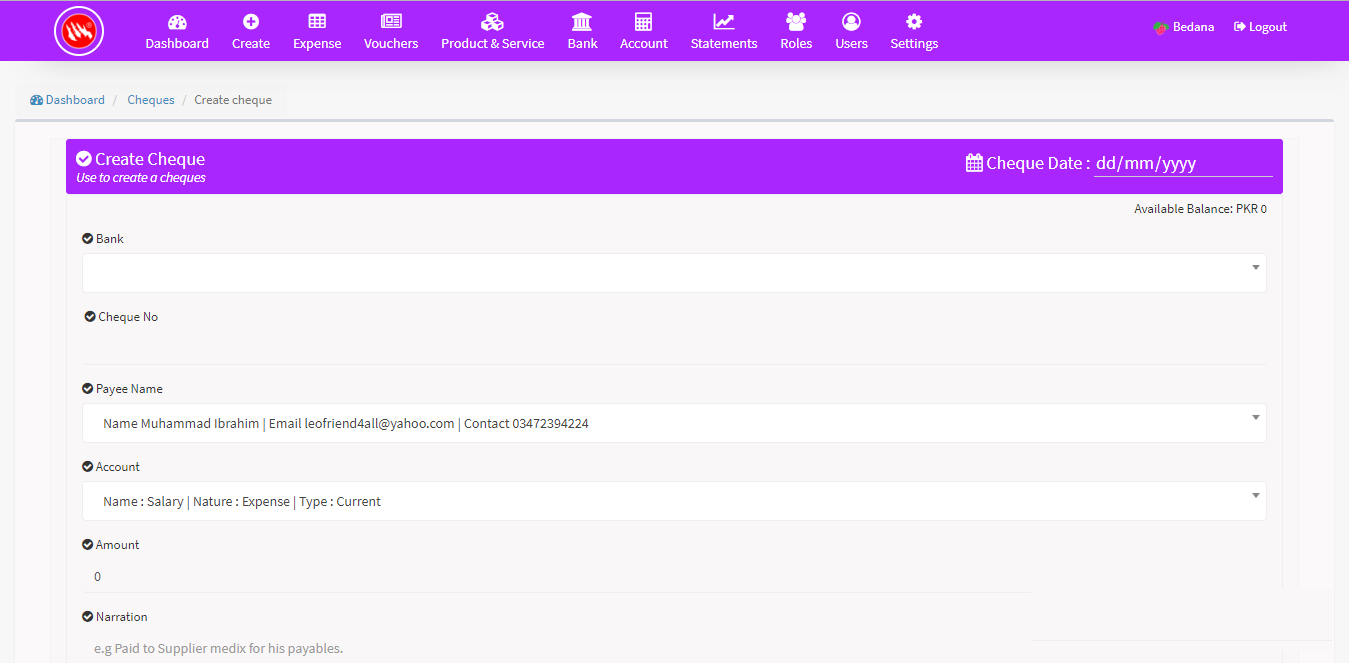In the image, there is a rectangular interface with the long side extending from left to right. Across the top of this rectangle is a prominent purple banner. On the far left within this banner, there is a red circle outlined in purple. As you move towards the right, several icons and words appear in a list, all rendered in white. These include: "Dashboard," "Create," "Expense," "Vouchers," "Product and Service," "Bank," "Account," "Statements," "Roles," "Users," and "Settings."

On the right-hand side of the purple banner, there is some unreadable text followed by either "logged in" or "logged out." Below this top banner, there is another banner displaying "Dashboard," "Checks," and "Create Check," with "Dashboard" being highlighted in green. A thin gray line runs horizontally beneath this second banner.

Further down, there is a third purple banner labeled "Create Check." This banner indicates its purpose: a form used to create a check. It includes several labeled fields: "Check date" with a placeholder DD/MM/YYYY, "Bank" with an open text box, "Check number," "Payee name" with an open text box, "Account" with another fillable box, "Amount," and "Narration."

Just beneath the third purple banner, there is a line of text indicating "Available Balance PXR0."